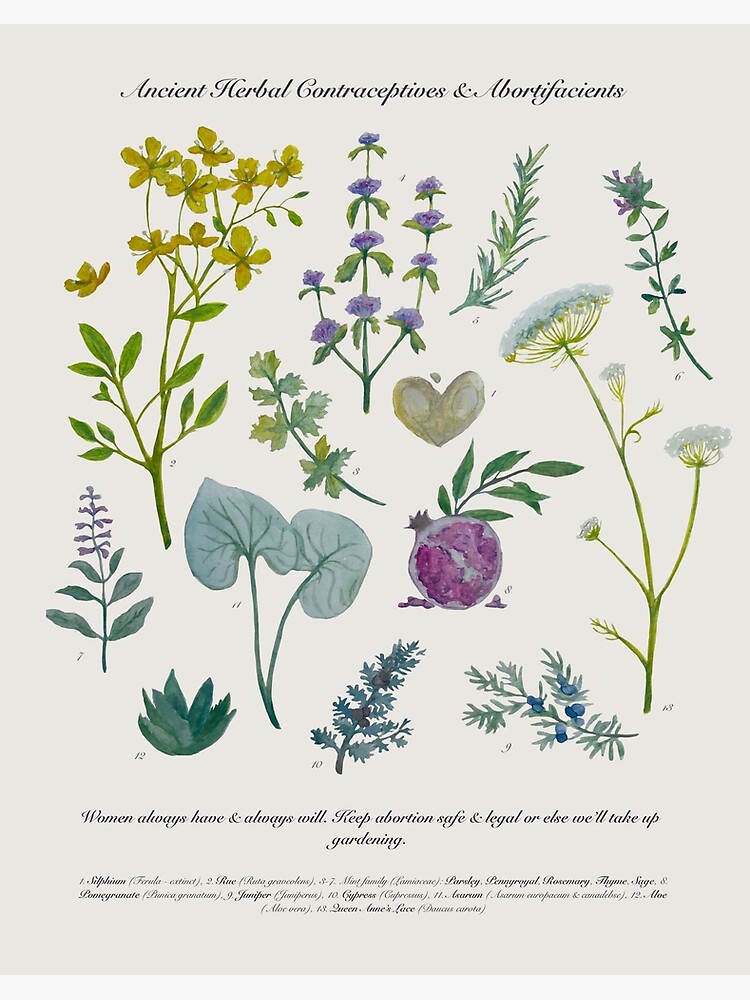The image is a detailed scientific identification diagram titled "Ancient Herbal Contraceptives and Abortifacients," presented in elegant cursive black text. It features 17 meticulously arranged drawings of various plants and herbs, including ferns, roots, flowers, and spices such as parsley, rosemary, thyme, sage, and pomegranate. The plants display a spectrum of colors—purple, green, gray, light brown, light gold, and white flower tips—against a grayish gradient background that enhances their visibility. At the bottom, a bold statement reads, "Women always have and always will keep abortion safe and legal, or else will take up gardening." Supplementary text, too small to read clearly, likely provides the genus and species names and additional information for each illustrated plant. The overall presentation aims to assert a political stance advocating for the legality and safety of abortion.